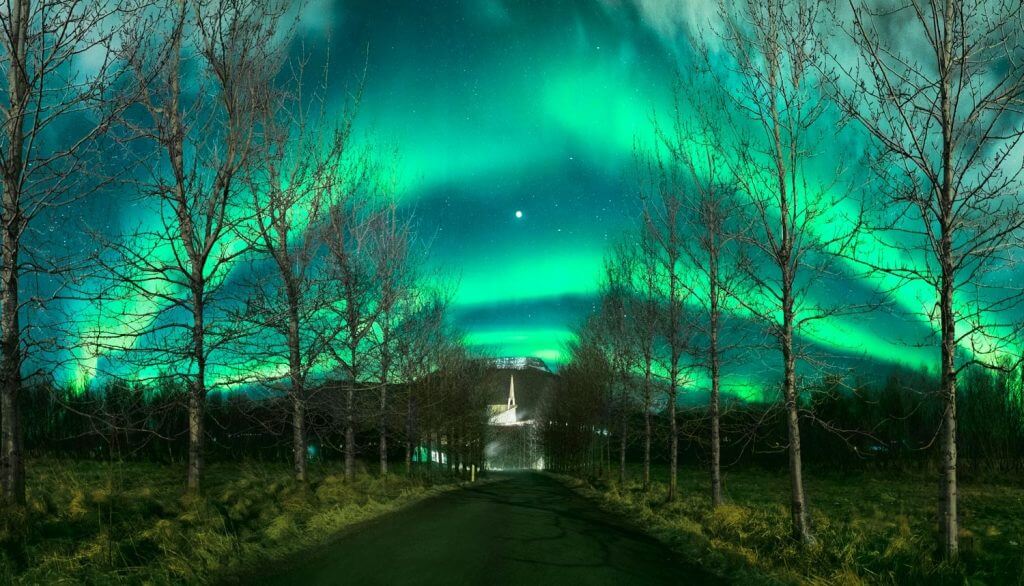This stunning horizontal digital illustration captures a serene night scene on a blacktop road, flanked by delicate, thin-branched trees. The road stretches into the distance, culminating in a bright, mysterious light source that appears to emanate from a building illuminated by streetlights or a spotlight. Behind this building, a dark hill rises, crowned by a distant mountain or structure. The sky above is the true spectacle, showcasing the ethereal beauty of the northern lights, which streak across the heavens in vibrant neon greens and blues. Stars twinkle in the center of the image, directly above the illuminated building, while light, fluffy clouds and wisps delicately intermingle with the celestial display.